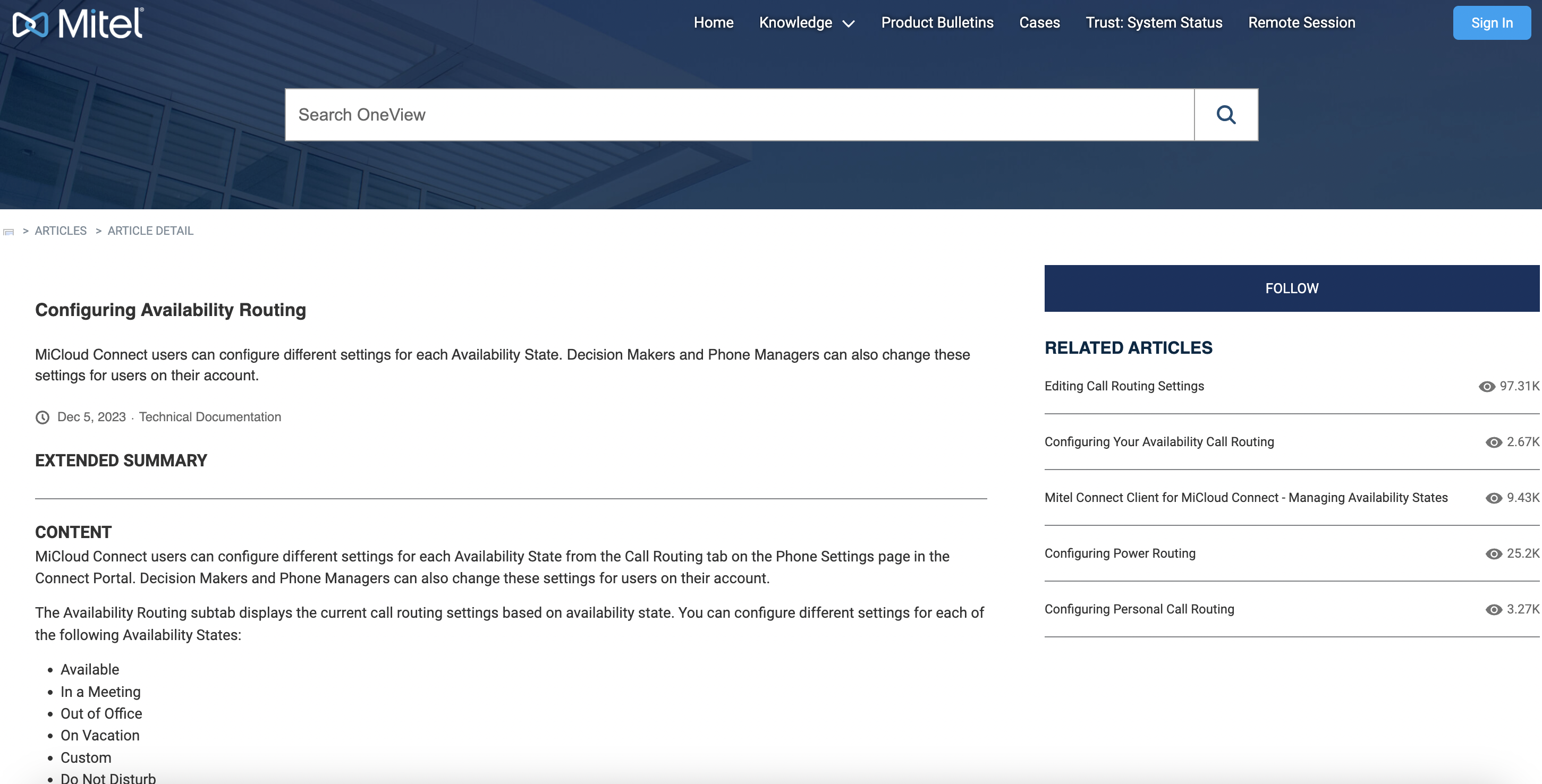The screenshot depicts a desktop or laptop interface with an elongated width characteristic of a computer monitor. The main background is predominantly white, adorned with black text. The top section features a blue-tinted header with a semi-transparent overlay of what appears to be the underside of a house overhang accompanied by windows.

In the upper left corner of the blue header, there's an icon resembling an hourglass turned on its side, followed by the text "Mitel" in white letters. Adjacent to this logo, a long white search box is prominently displayed, bearing the placeholder text "search oneview"—indicating the name of the search function.

The interface is partitioned with tabs, clearly showing that the current view is set to "article details." The main content area below this header begins with the heading "Configuring Availability Routing," followed by an "Extended Summary" section. To the right-hand side of this main text block, there is a sidebar featuring a list of links to related articles, providing additional resources and information on related topics.